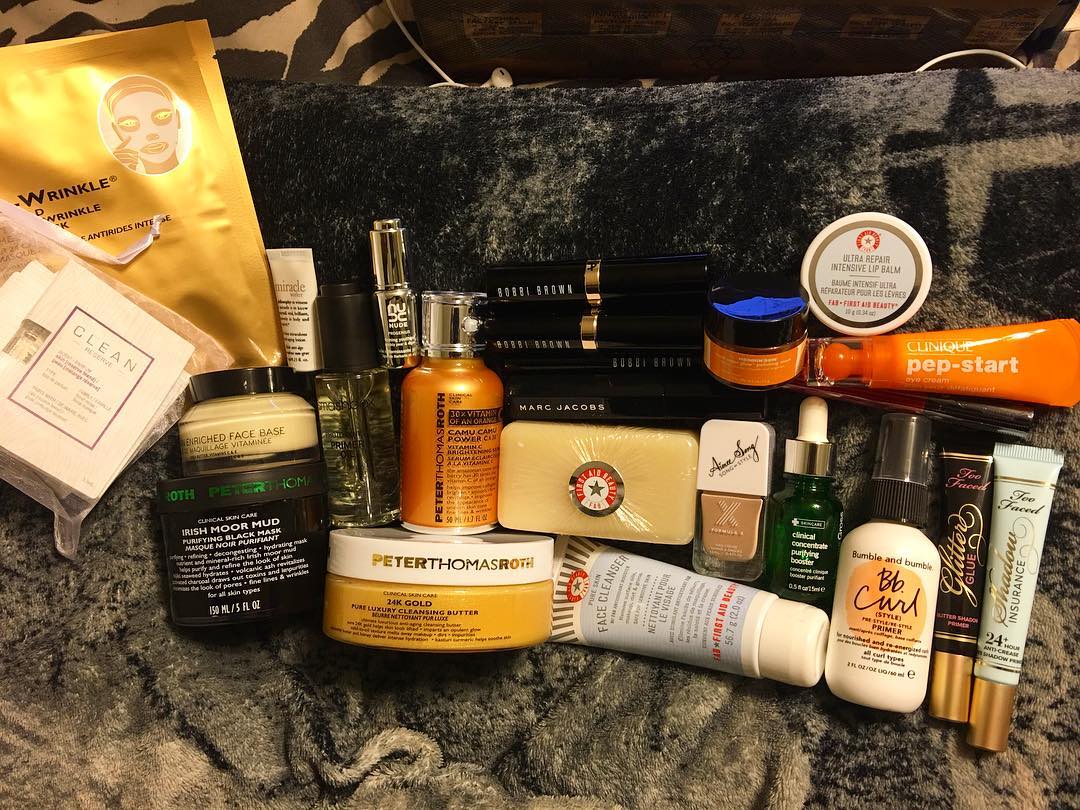The image features a carefully arranged assortment of beauty products displayed on a plush blanket. Dominating the backdrop is a zebra print blanket situated in the top left corner. A box occupies the upper right section of the image, casually accompanied by a set of headphones with their cords neatly tucked away behind it. Draped across this scene is another luxurious blanket, its texture and hues ranging from black to a soft light gray, adding a touch of elegance.

In the foreground, a variety of beauty products are meticulously aligned, offering a glimpse into diverse skincare and cosmetic regimens. From left to right, the featured items include:

1. A wrinkle mask encased in a shimmering gold pouch.
2. A "Clean Serum" housed in a white mesh pouch.
3. A small jar labeled "Enriched Face Base."
4. A plastic tub branded "Irish Moor Mud."
5. A compact white tube marked "Miracle."
6. A clear glass dispenser with unreadable text.
7. A minuscule dispenser inscribed with "Nude."
8. A copper-colored bottle labeled "Camu Camu Powder."
9. A squat, gold and white jar that reads "Peter Thomas Roth 24 Karat Gold Cleansing Butter."
10. Three mascara tubes with the brand "Bobbi Brown" and one mascara tube labeled "Marc Jacobs."
11. A square soap bar.
12. A tube labeled "Face Cleanser."
13. Formula X nail polish.
14. A green dropper bottle marked "Clinical Concentrate Purifying Booster."
15. A white spray bottle labeled "BB Curl."
16. Two tubes: one reading "Glitter Glue" and the other "Shadow Insurance."
17. A small orange tub with unreadable text.
18. A small white tub labeled "Ultra Repair Intensive Lip Balm."
19. An orange tube bearing the label "Clinique Pep-Start."

This precise collection of beauty products offers a rich tapestry of skincare solutions, brilliantly captured in an organized yet organic tableau.